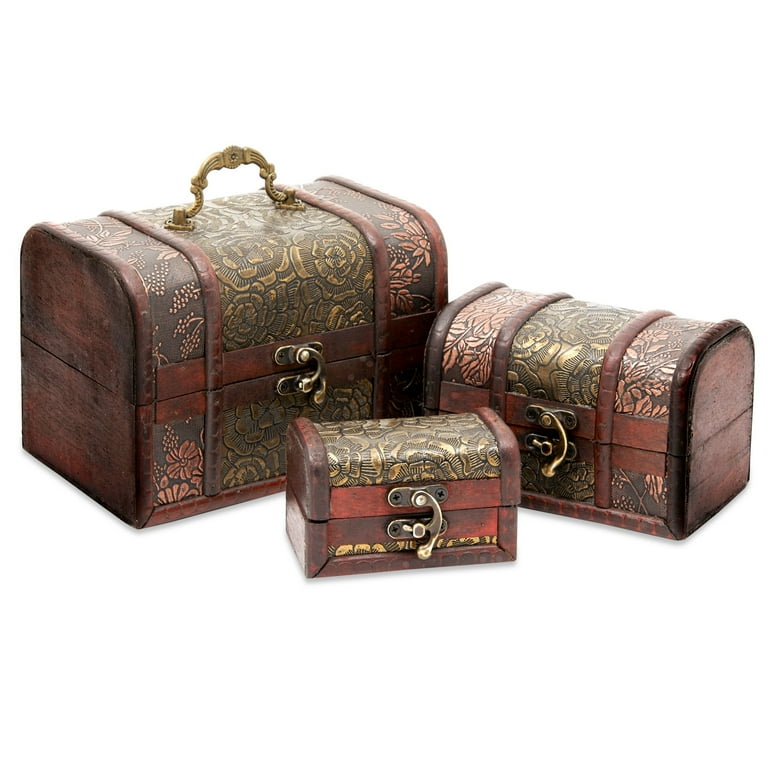This is a photograph of an ornate set of old-fashioned luggage comprised of three pieces, each resembling antique wooden chests with rectangular shapes and rounded edges. The chests are crafted from what appears to be dark-stained wood, embellished with gilded inlay or embroidering on their surfaces, which adds to their vintage charm. The largest chest, designed to be carried like a suitcase, features a decorative brass handle and a hasp that clasps onto the bottom. The second chest, approximately half the size of the largest, shares the same intricate design but lacks a carrying handle. The smallest piece, possibly a jewelry box, mimics the elaborate style of the larger two and is akin to a handbag in size. Together, these nested pieces create an elegant ensemble of matching, antique-style luggage.